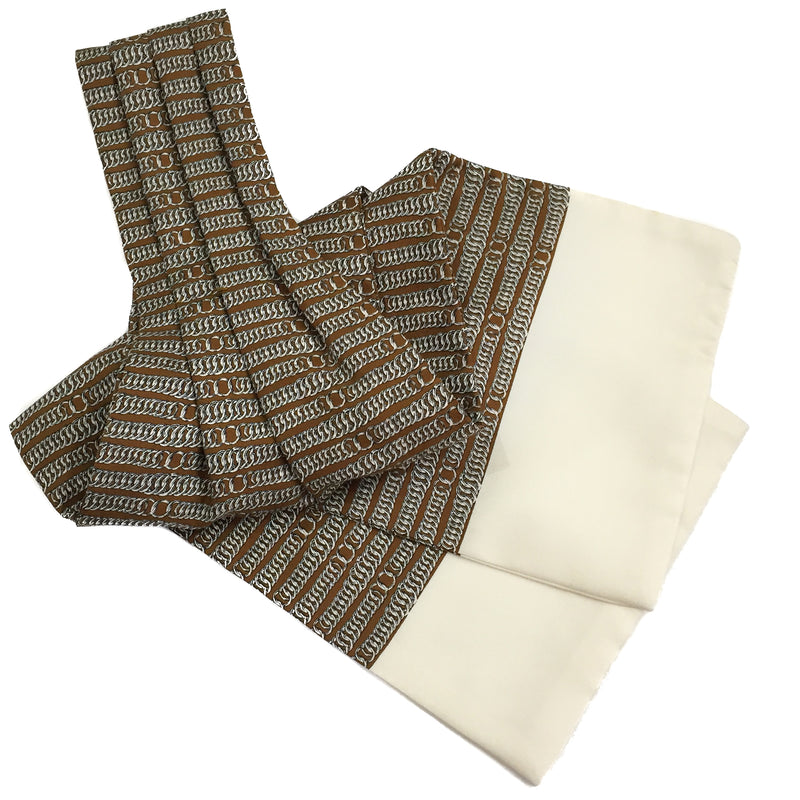This square image presents a detailed view of a piece of fabric, possibly a scarf, set against a completely white background without any borders. The fabric, primarily brown with a twill pattern, features horizontal gray or silver chain-like stripes running across it. On both ends of the fabric, there are prominent beige border trims that might be made of cotton or linen, providing a distinct edge to the piece.

In the bottom right corner, the fabric is folded over itself, creating a rectangular overlapping section with the top piece tilted and angled upwards to the right. This folding arrangement, combined with the beige trimmed edges, almost gives an impression of socks but it's clearly not. Towards the upper left corner of the image, the fabric gathers into pleats, which emphasizes the chain pattern continuing consistently through the folds.

The photograph is devoid of any labeling or writing, highlighting the material and design without distraction.